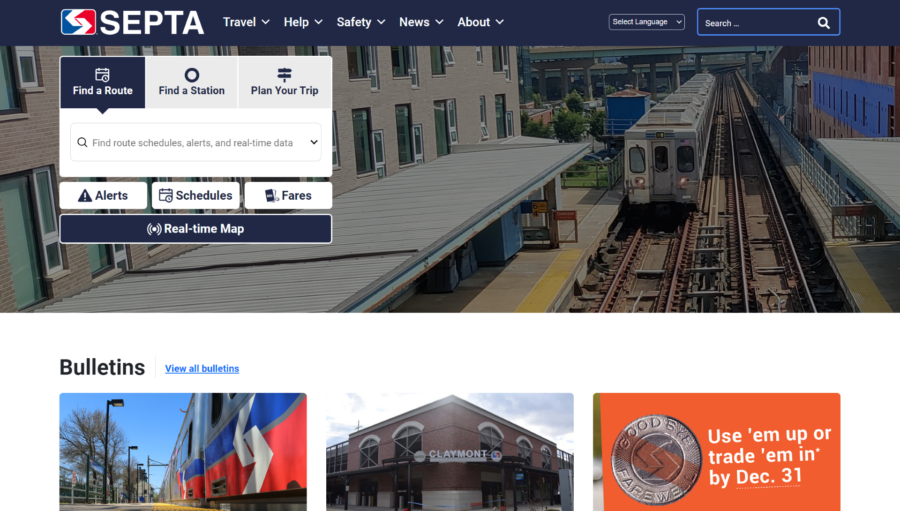The image appears to be a screenshot of a travel-related website, likely the homepage, featuring a detailed layout and branding associated with SEPTA. In the top left corner, there is a SEPTA logo consisting of red, white, and blue colors in a geometric square design, accompanied by "SEPTA" in white text. This section of the website includes several navigation buttons labeled 'Travel', 'Health', 'Safety', 'News', and 'About', all of which have drop-down menus indicated by downward arrows.

A blue border runs across the top of the page, encompassing the aforementioned buttons, with 'Select Language' and a medium-sized search box labeled 'Search' located towards the right side. The background photo spans across the top of the page and depicts a train traversing tracks in what looks like a subway or train station, with buildings and an overpass visible in the background, suggesting it might be a commuter train.

Superimposed on the photo is a user input form designed for travel planning. It includes interactive elements like buttons for 'Find a Route', 'Find a Station', and 'Plan Your Trip'. Additionally, there is a real-time map feature and clickable photo buttons labeled 'Bulletins', indicating travel-related updates and bulletins.